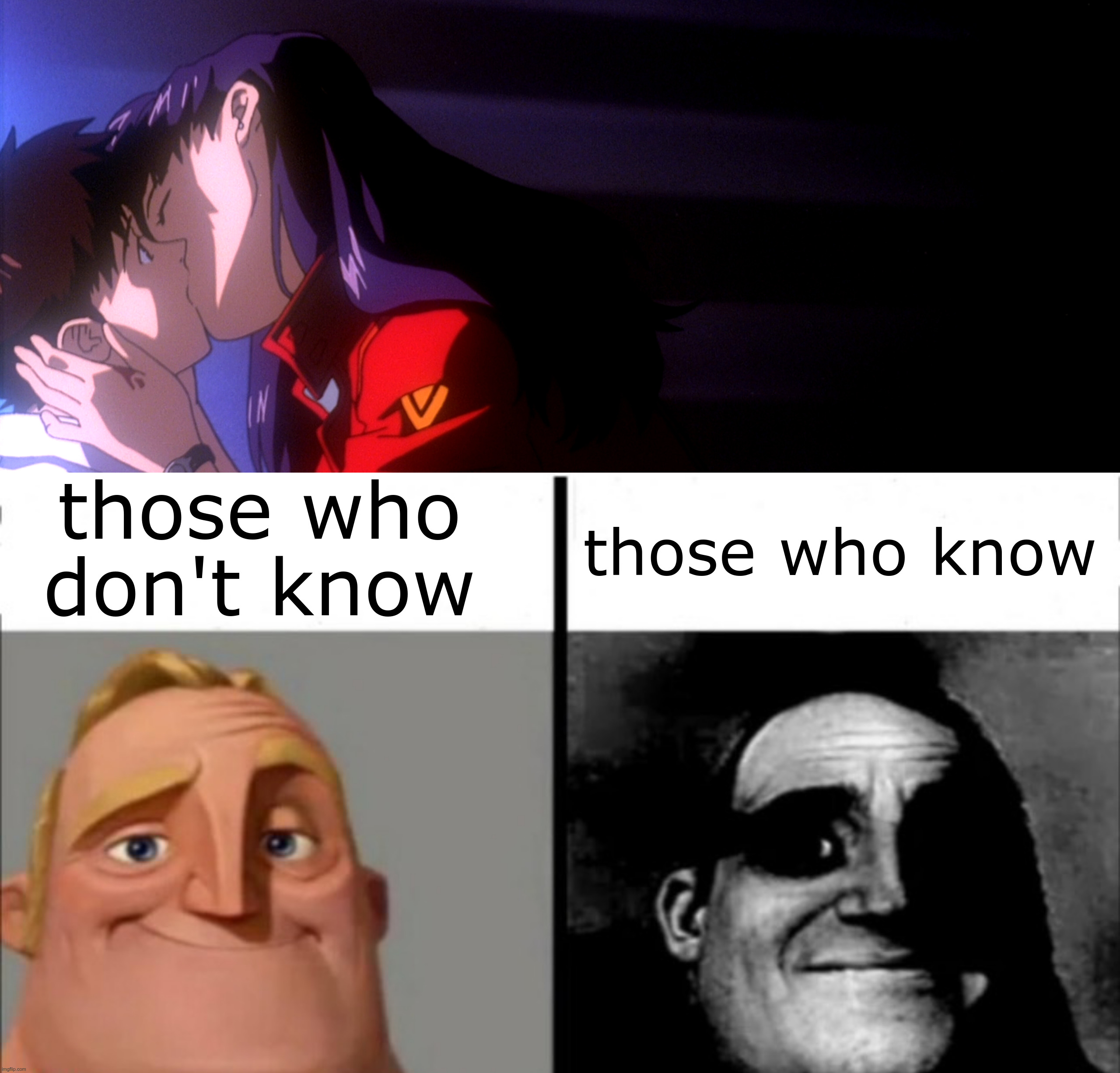The given image is divided into three sections. At the top, it features a colored illustration of two people kissing. The woman, located on the left side of this segment, has long purple hair and is wearing a red top. She also has some sort of device on her left wrist. The man, positioned to her right, has black hair and his eyes are open, while the woman's eyes are closed.

On the bottom left section of the image, there is a caption that reads "Those who don't know," written in black text. Below this caption is an artistic depiction of a man's face with blonde hair, blonde eyebrows, and blue eyes. He is smiling and his ears are visible. The background is gray with no other details.

The bottom right section has the caption "Those who know." Below this text is a black and white illustration of the same man's face as depicted on the left. No other elements are present in the background.